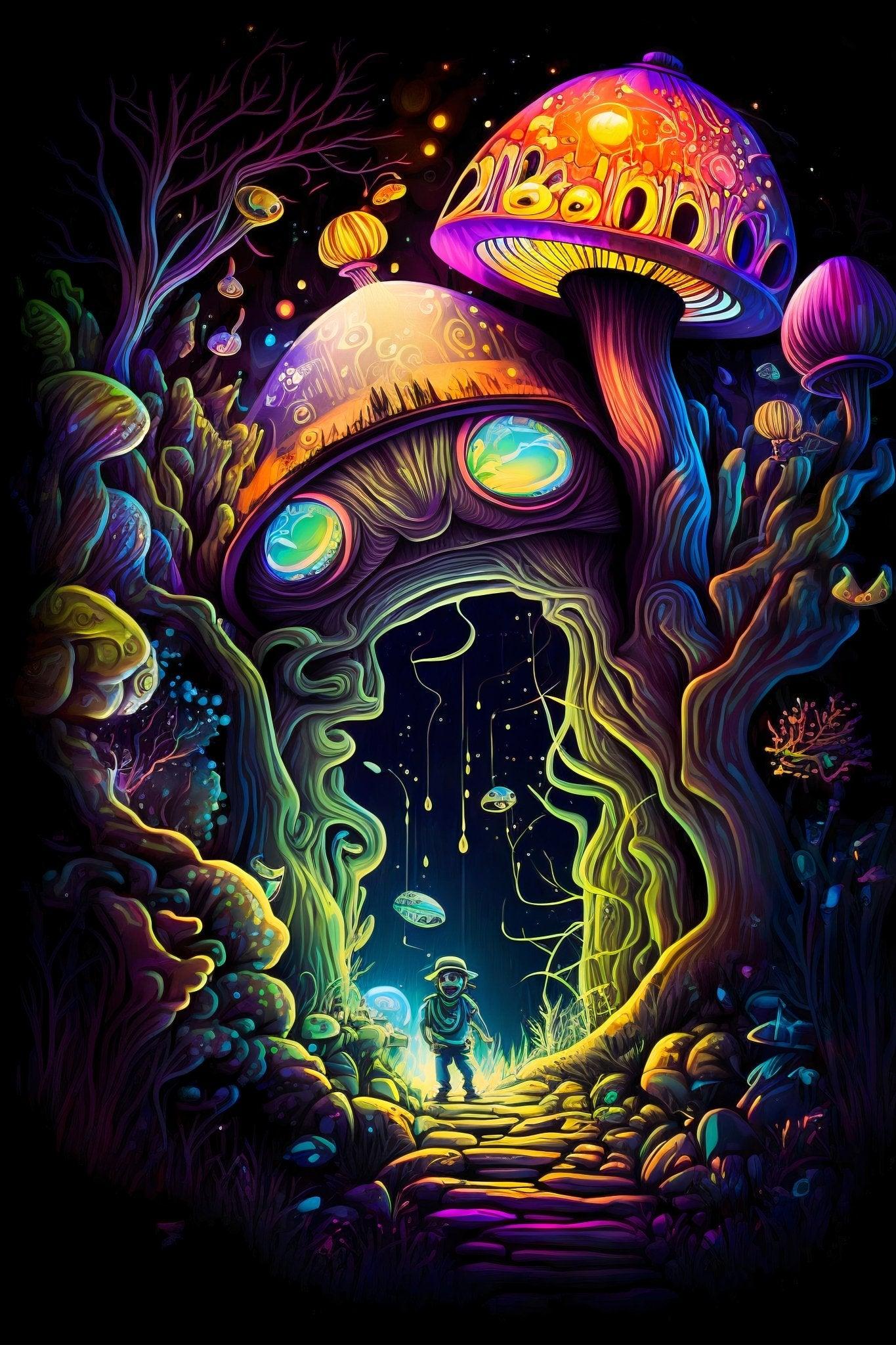In this vibrant and psychedelic artwork set against a black background, a captivating scene unfolds. The central feature is a hollowed-out log or stump, from which two wavy branches morph into large mushroom caps. The main stump has circular eyes framed in neon purple, with lenses that blend green, yellow, and blue hues. Its open mouth forms an archway, emitting an ethereal glow, under which a small human figure dressed in a hat, t-shirt, and jeans walks along a rocky, cobblestone path.

Above this archway, otherworldly and vivid mushrooms sprout. One towering mushroom has a red cap with a ring of holes and a yellow, veiny underside. The stalk of this mushroom, like others around it, is textured and robust. The scene is brought to life with glowing fireflies, blue orbs, and descending elements resembling shooting stars. Delicate, spaghetti-like appendages dangle from the stump's center, each ending in a neon-yellow teardrop. The use of bright pink, purple, blue, and green colors against the dark backdrop further enhances the enchanted, dreamlike atmosphere of this mushroom forest.